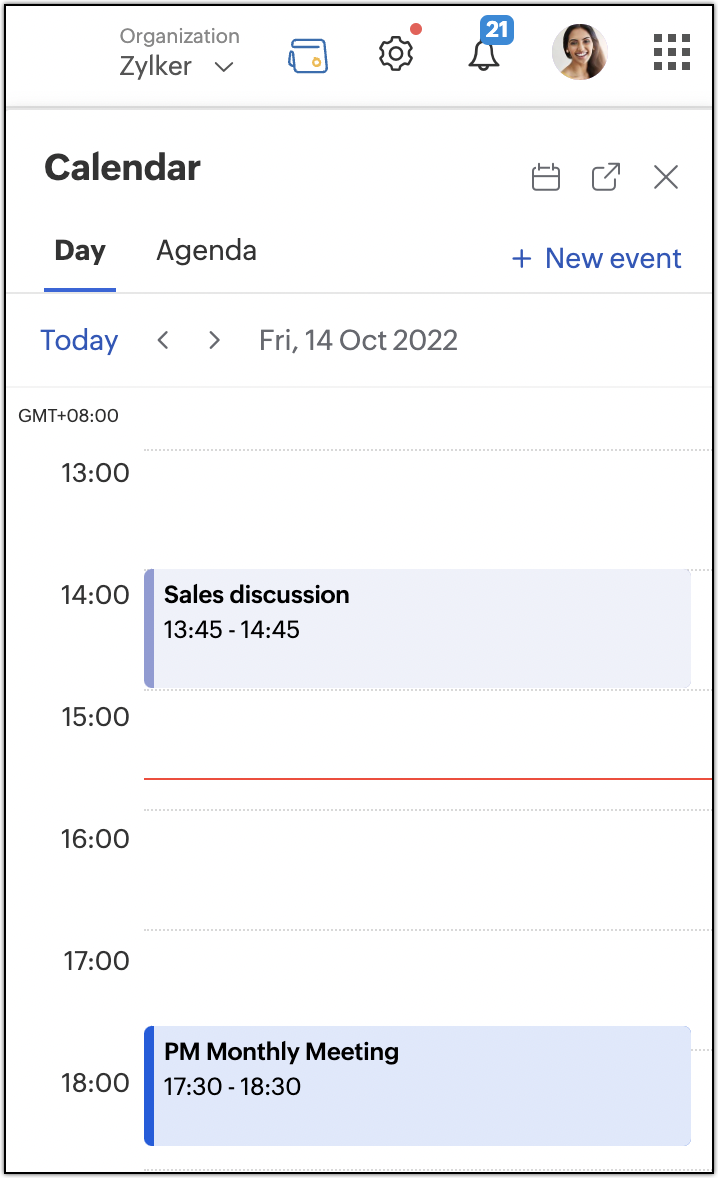This screen capture displays an interface with a white background and primarily black text, bordered by a thin black line. At the top, the name "Zylker" (Z-Y-L-K-E-R) is shown alongside a dropdown arrow. Below it, a series of icons appear on the right side of the screen: a blue outlined credit card icon with a gold dot, a black cogwheel icon with a red dot, a black bell icon with a blue box containing the number 21 in white, and a circular photo of a smiling woman with brown hair.

On the left-hand side, a series of gray squares can be seen, leading down to a menu that lists "Calendar." Within the calendar section, options for viewing schedules by "Day" and "Agenda" are displayed. There's a blue button labeled "New Event" next to several icons, including a calendar icon, a square with an arrow, and an 'X' icon.

Under the "Day" section, the current date "Today," Friday, October 14, 2022, is highlighted in blue. The timezone is noted as GMT +8. Various scheduled times are displayed below:

- 13:00
- 14:00
- A blue box indicating "Sales Discussion," scheduled from 13:45 to 14:45
- A red flat line from 15:00 to 16:00
- A gray line from 16:00 to 17:00
- A blue box indicating "PM Monthly Meeting," scheduled from 17:30 to 18:30

These details are presented in an organized manner, allowing the user to manage their schedule effectively.